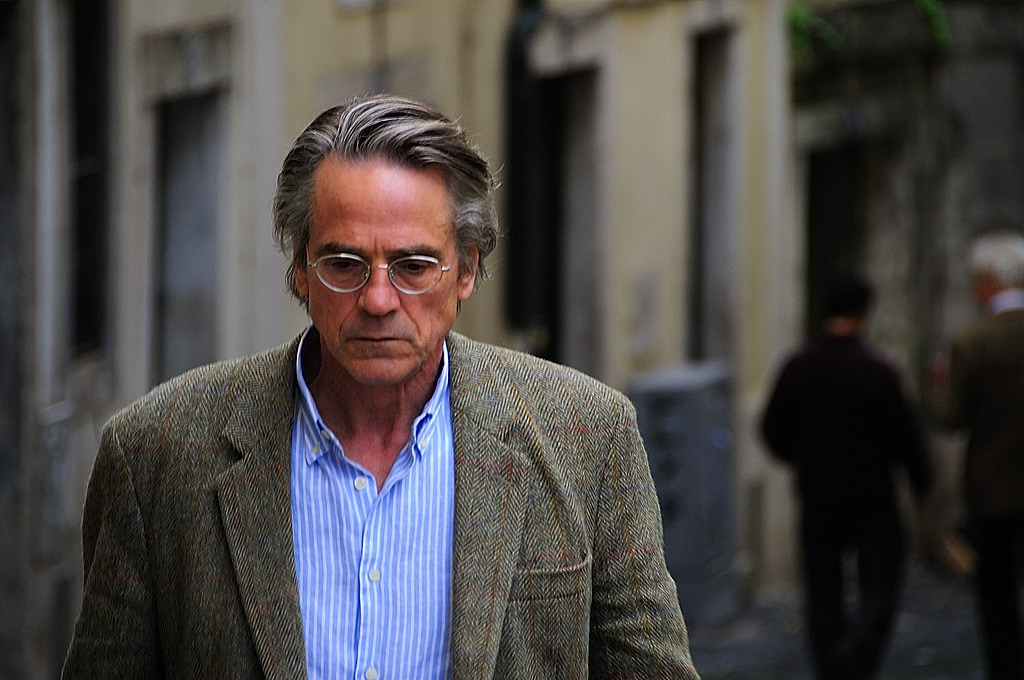The image features actor Jeremy Irons, a Caucasian man likely in his late 40s to early 50s, captured from his lower chest up. Irons sports a contemplative expression, looking downward, with thin-framed silver glasses resting on his face. His hair, a salt and pepper mix, is styled back with a slight wave to the side, indicating minimal use of hair gel. He is dressed in a tweed, dark grayish-green to light brown jacket over a collared button-up dress shirt adorned with vertical light blue and white stripes. The top button of his shirt is casually undone. Behind him, the background appears blurred, revealing an indistinct concrete-colored building and two men walking away toward the right; one dressed in black and the other in a suit with a white collar. The scene suggests a film set or a staged setting, with an overall focus on Irons' serious demeanor.